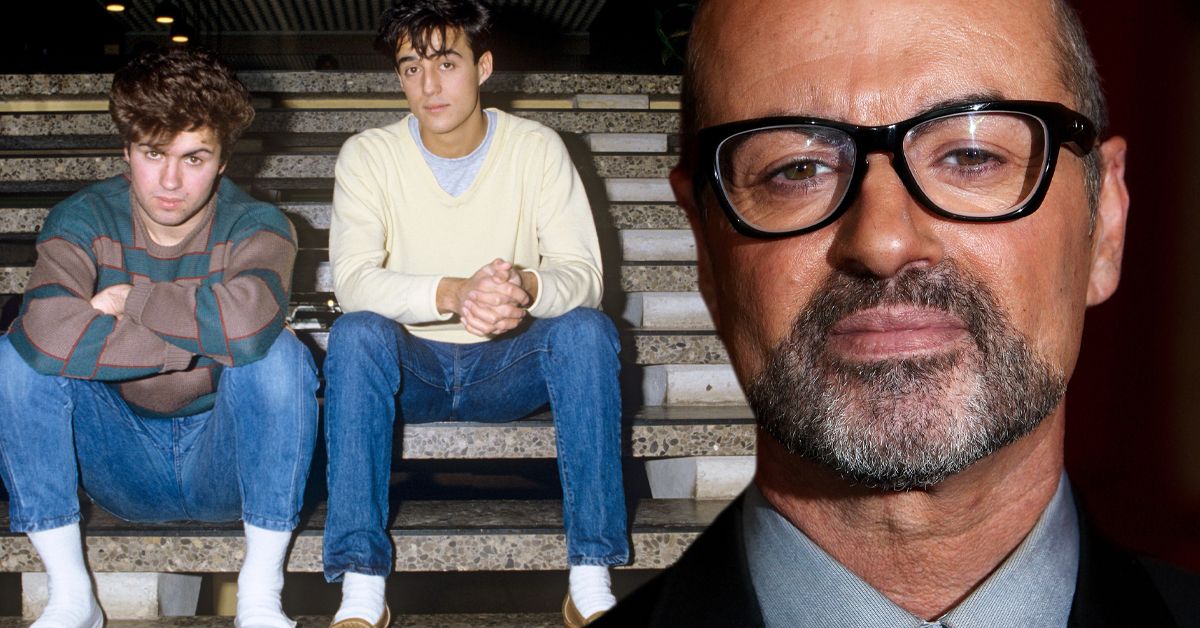The image is a horizontally aligned rectangular picture featuring three individuals. On the left, two young men are seated on a staircase. The man on the bottom stair resembles a young George Michael, with short, very curly longer hair on top, dressed in blue jeans and a striped brown and green top, with white socks. He sits with his arms crossed and elbows resting on his knees. Next to him, slightly elevated on the staircase, is another young man, possibly a band member, wearing blue jeans and a light yellow or beige sweater with long brown hair falling over his forehead. Both young men have their hands clasped together, leaning on their knees. On the right side of the image is a close-up of an older man who may also be George Michael. He has black-rimmed glasses, a very short salt-and-pepper beard, and wears a collared gray shirt under a dark suit jacket. Only the top of his shoulders and part of his head are visible in the close-up. The overall image appears to document a passage of time, highlighting the contrast between the youthful and older appearances of the subjects, possibly suggesting a before-and-after narrative.